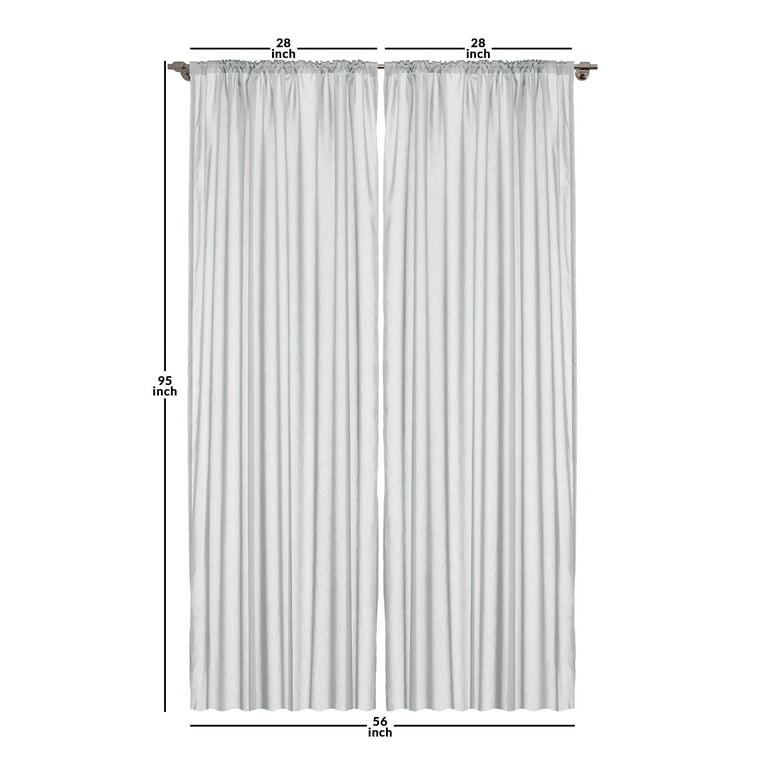This product photograph showcases a set of two light gray, floor-length curtain panels, neatly hung from a mounted silver metal curtain rod. The background is a pristine, solid white to ensure complete focus on the product. Each curtain measures 28 inches wide, making the total combined width 56 inches, as indicated by black text on horizontal lines above and below the curtains. A vertical line on the left side of the image marks the length of the curtains at 95 inches from top to bottom. The image, likely intended for use in online listings such as catalogs or e-commerce websites, meticulously highlights these dimensions to provide clear and detailed information to potential buyers.